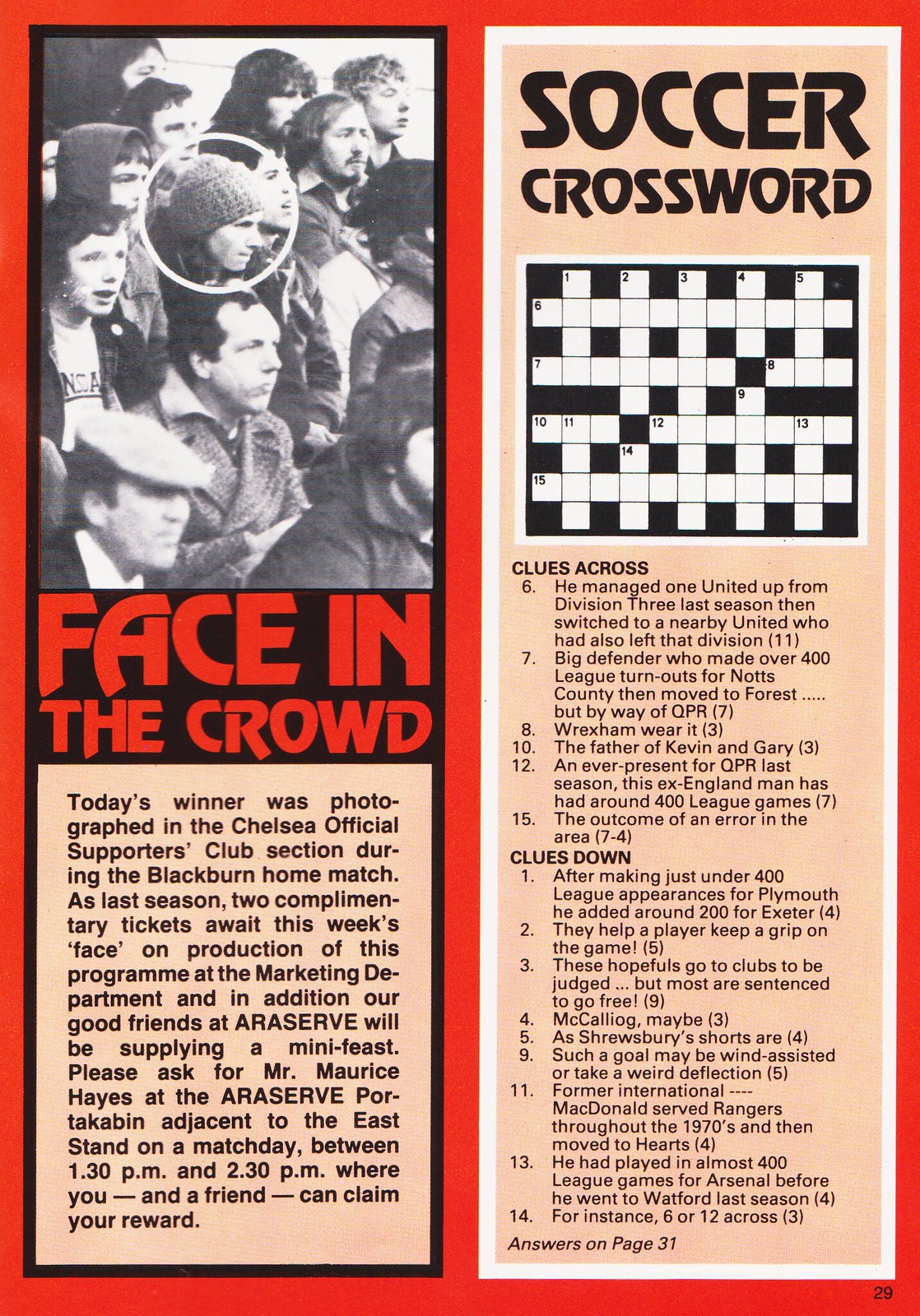This image appears to be a page taken from a game program or magazine, split into two distinct halves. On the left, there is a black-and-white photograph of a crowd, with a red-font title "Face in the Crowd." Among the spectators, a man wearing a beanie hat is circled, indicating he is the highlighted individual. Below the photograph, a detailed write-up announces the man as the winner, photographed in the Chelsea official supporters club section during the Blackburn home match. Winners receive two complimentary tickets upon presenting this program at the marketing department. Additionally, AeroServe provides a mini feast, redeemable by asking for Mr. Maurice Hayes at the AeroServe port cabin adjacent to the East Stand on match days between 1:30 PM and 2:30 PM.

On the right side of the image, there is a soccer-themed crossword puzzle set against a peachy-orange background. The crossword is not filled out and includes both across and down clues. The answers are stated to be available on page 31.